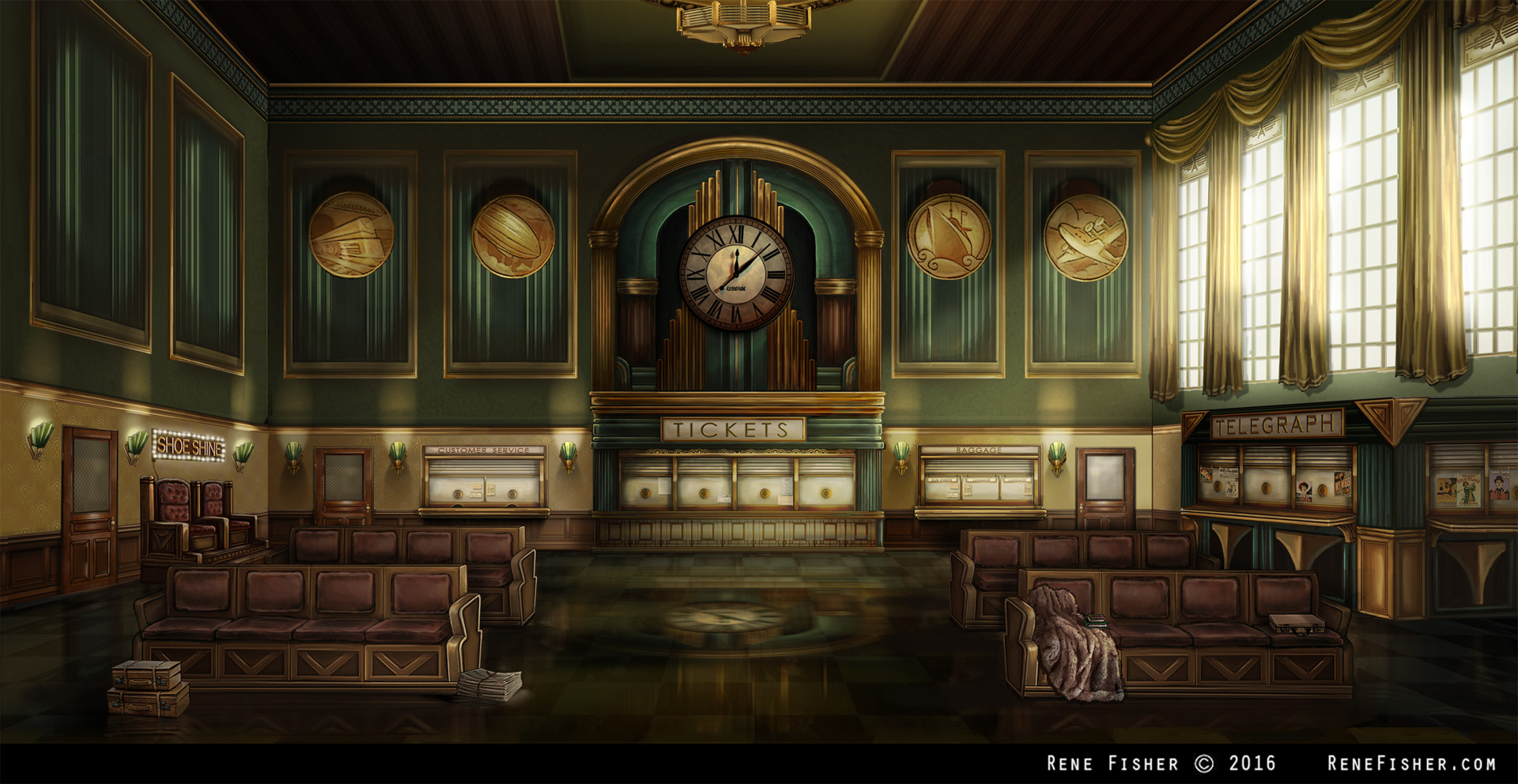This detailed image appears to be an intricate, possibly computer-generated artwork of an old-fashioned train station. The large room is bathed in natural light coming from big windows on the right-hand side, which are adorned with white curtains. The walls are decorated in green and gold, exhibiting various photographs and metal images highlighting different modes of transportation, including trains, planes, and boats. Centrally positioned on the back wall is a large, round clock with Roman numerals, displaying the time as approximately 12:10. Directly beneath the clock is a sign that reads "Tickets." 

To the left of the clock are designated areas for "Customer Service" and "Baggage." Meanwhile, on the far right, a sign indicates the "Telegraph" office, and on the left-hand side of the room, there is a lit-up sign for "Shoeshine" next to two chairs. Further adding to the nostalgic charm, golden emblems are hanging on the walls, and several rows of benches are placed throughout the space. One bench has a mink coat and a hat draped over it, while another has a blanket. The piece is signed "Renee Fisher 2016" at the bottom, with a reference to the artist's website, reneefisher.com.